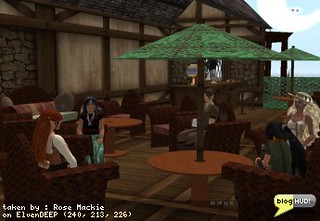In this video game-inspired image, a group of characters is seated in a vibrant, outdoor setting under a green umbrella-topped table. The ensemble includes a woman with striking orange-red hair, another with vivid blue hair, a man casually sitting in a wicker chair, and a blond-haired woman situated to the right. Another woman, also seated in a wicker chair, completes the group. Captured by Rose Mackey on 11 Deep, 240-213, Blog HUD, the scene evokes the ambiance of popular life simulation games like The Sims or Minecraft.

The background features a wooden structure, giving off the vibe of a cozy, open-air restaurant. There are additional orangish-brown tables and unoccupied wicker chairs, suggesting a lively gathering space. Behind the tables, a bar area and a green gate are visible, framed by a light blue sky that enhances the outdoor setting’s charm. The meticulous details and vibrant colors contribute to an immersive and bustling environment typical of virtual community spaces.